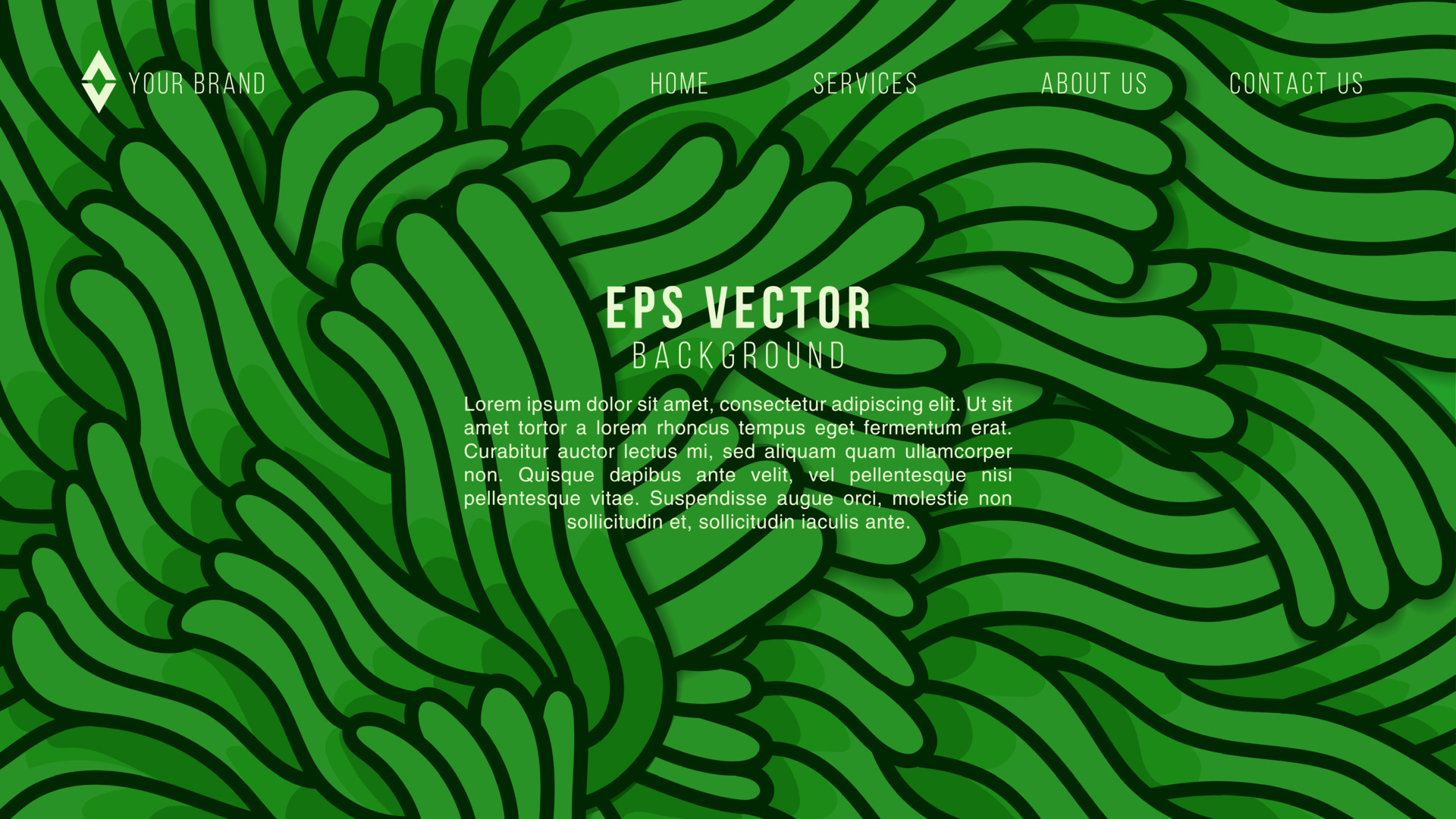A detailed depiction of the image, consolidating all provided descriptive elements, would be:

The image appears to be a mockup of a website template, portraying a potential homepage layout adorned with artistic green waves outlined in black, resembling playful seaweed or tentacle-like shapes spread across the entire rectangular frame. At the top left corner, it displays the placeholder text "Your Brand" with a set of triangles pointing up and down beneath it, establishing a central brand identifier. Across the top right section, there's a navigation menu comprising four tabs labeled "Home," "Services," "About Us," and "Contact Us." Dominating the center of the image is the text "EPS Vector Background" alongside an array of unreal or Latin words, signifying that this is a generic mockup template. The central and background artwork contributes a whimsical and artistic touch to the overall design.